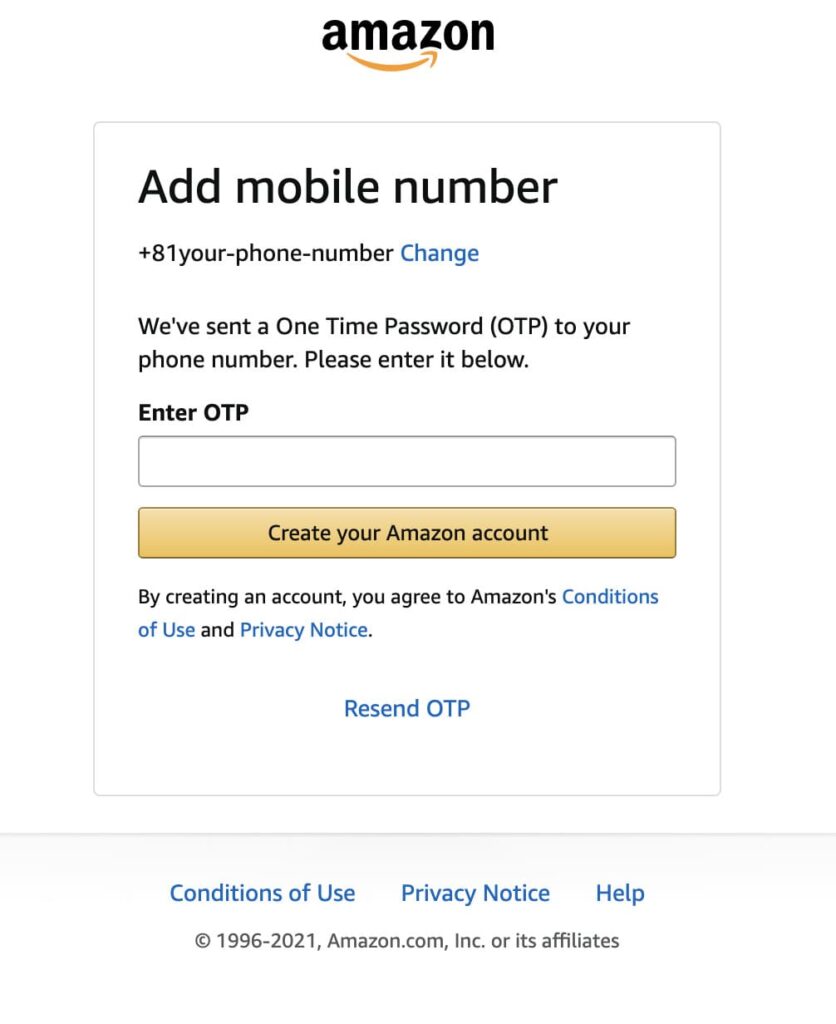This is a detailed screenshot of an Amazon AdMobile phone verification page. At the top center, there is the iconic Amazon logo set against a clean, white background. Directly beneath the logo, there's a rectangular box containing the text: "AdMobile number +81 [your phone number]. Change" in blue. 

Below this box, a message reads, "We've sent a one-time password (OTP) to your phone number. Please enter it below." Subsequently, there's an input field designed for users to enter their OTP.

Under this input field, an orange button prominently displays the instruction, "Create your Amazon account." Beneath this button, a line of text informs the user, "By creating an account, you agree to Amazon's Conditions of Use and Privacy Notice," with the phrases "Conditions of Use" and "Privacy Notice" highlighted in blue, indicating clickable links.

At the very bottom center of the image, a blue text link reads, "Resend OTP," offering users the option to request another password.

Outside the main content area, in the footer, there are three links arranged in a row that say "Conditions of Use," "Privacy Notice," and "Help." Finally, the footer includes a copyright notice: "© 1996-2021, Amazon.com, Inc. or its affiliates."